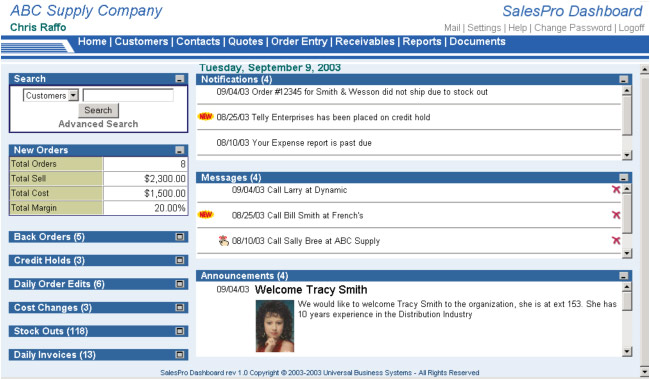The screenshot depicts a webpage from ABC Supply Company's SalesPro Dashboard, managed by Chris Raffo. The top right corner offers various user options such as Mail Settings, Help, Change Password, and Log Off. Directly below, a horizontal navigation bar showcases tabs labeled Home, Customers, Contact Quotes, Order Entry, Portables, Reports, and Documents, all set against a blue background with white font.

On the left side of the page, there is a search area designated for "Customers" with a dropdown menu and a white search field, accompanied by buttons labeled "Search" and "Advanced Search" beneath it. Further down, key performance metrics are displayed: "New Orders: 0," "Total Orders: 0," "Total Sale: $2,300," "Total Cost: $1,500," and "Total Margin: 20%." Additional logistical data includes "Back Orders: 5," "Credit Holds: 3," "Daily Order Edits: 6," "Cost Changes: 3," "Stock Outs: 118," and "Daily Invoices: 13."

On the right side of the webpage, the date is prominently displayed as "Tuesday, September 9, 2003." Below this, notifications specify that on September 4th and August 25th, certain orders encountered issues: the orders for Smith and Wilson did not show up due to stockouts on 9-4-3, and Tele Enterprises has been placed on credit hold on 8-25-3.